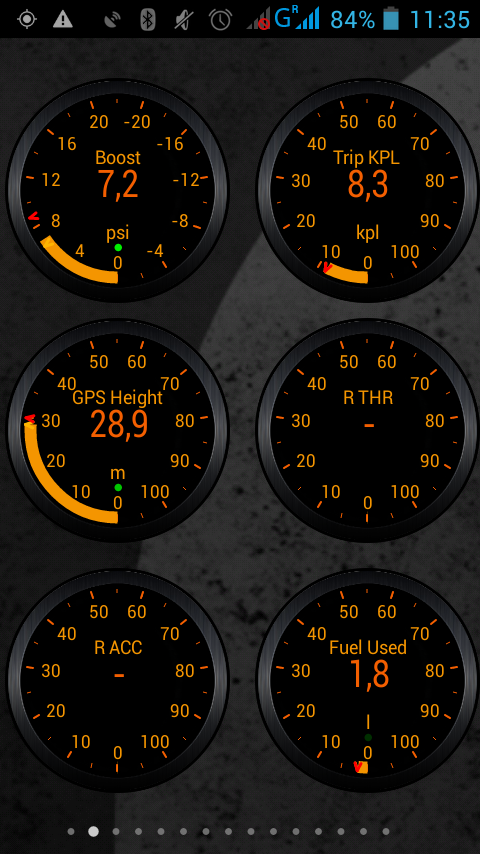The image is a detailed screenshot from an Android phone showing the status bar at the top with various icons, including Bluetooth, geolocation, mute, signal strength, and battery status at 84%. The time displayed in the top right corner reads 11:35. Below the status bar, the main content of the screen features six skeuomorphic dials with a 3D appearance, arranged in three rows and two columns. Each dial has a black background with yellow numbers around it, orange ticks, and central orange values. The first dial, labeled "Boost," shows a reading of 7.2 PSI. The second dial, labeled "Trip KPL," reads 8.3 and is measured in kilometers per liter. The third dial, "GPS Height," displays 28.9 meters. The fourth dial, "RTHR," has no specified measurement. The fifth dial, "RACC," also has no measurement indicated. The sixth and final dial, labeled "Fuel Used," shows 1.8 liters.